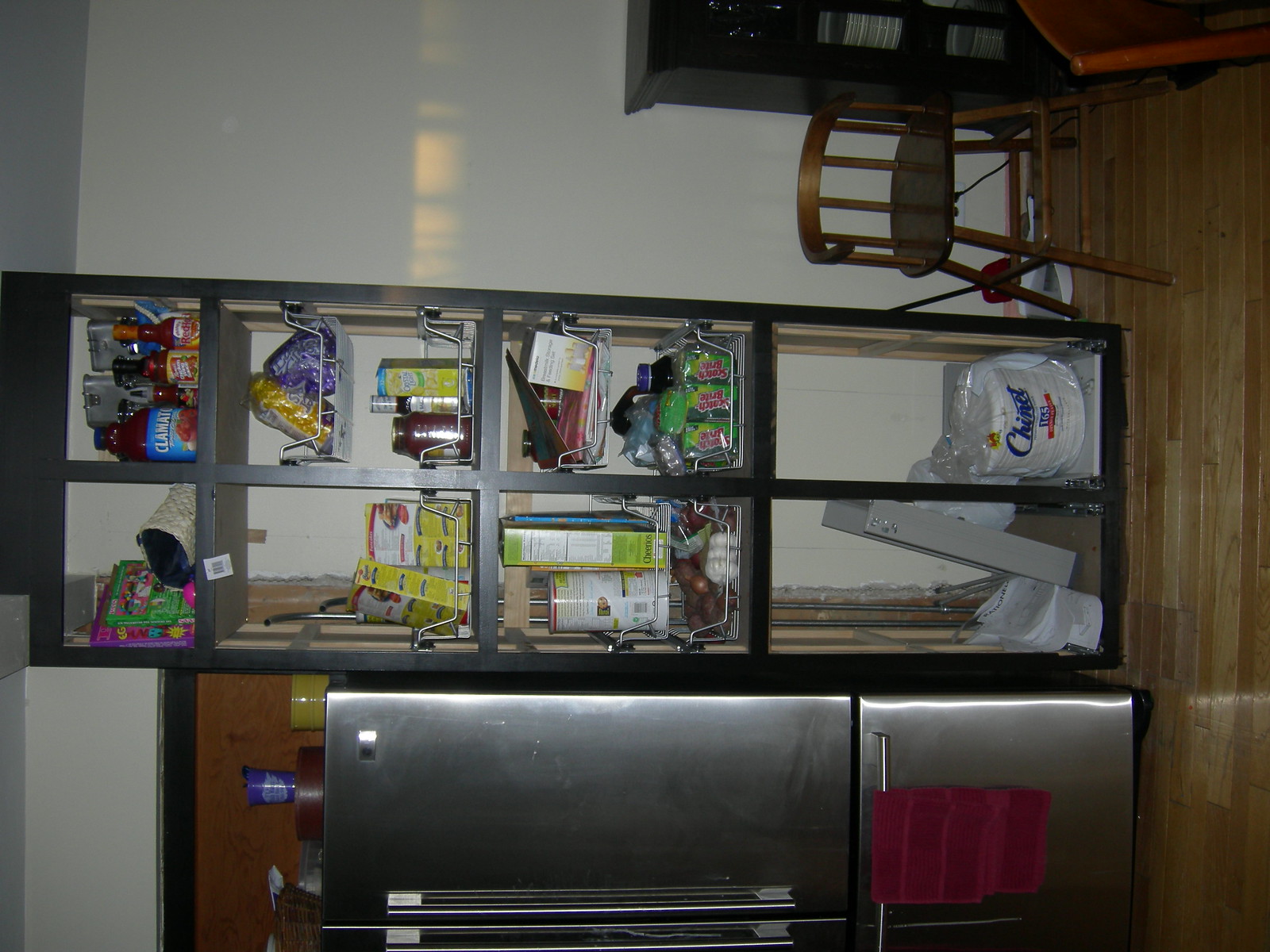This photograph captures a kitchen that is currently oriented 90 degrees to the left, but I'll describe it as if it were upright for better clarity. In the middle of the left-hand side stands a sleek, four-sectioned silver refrigerator. The upper two sections serve as the refrigerator, while the bottom two sections appear to be freezer drawers, one of which has a towel draped over it. The refrigerator is positioned on a wooden floor, directly in front of what resembles a door frame, with an orange wooden panel situated behind it.

To the immediate right of the refrigerator, there is a tall, floor-to-ceiling shelving unit that serves as an informal pantry. This unit is packed with a variety of items, including baskets, boxes, cans, bottles, paper plates, and brushes, creating a sense of organized chaos. 

Additionally, there is a small chair next to the shelving unit, which appears to be elevated and possibly designed for a child. Finally, to the right of this chair at the base of the back white wall, the first foot or so of a bookcase is visible, hinting at further storage or decorative items.